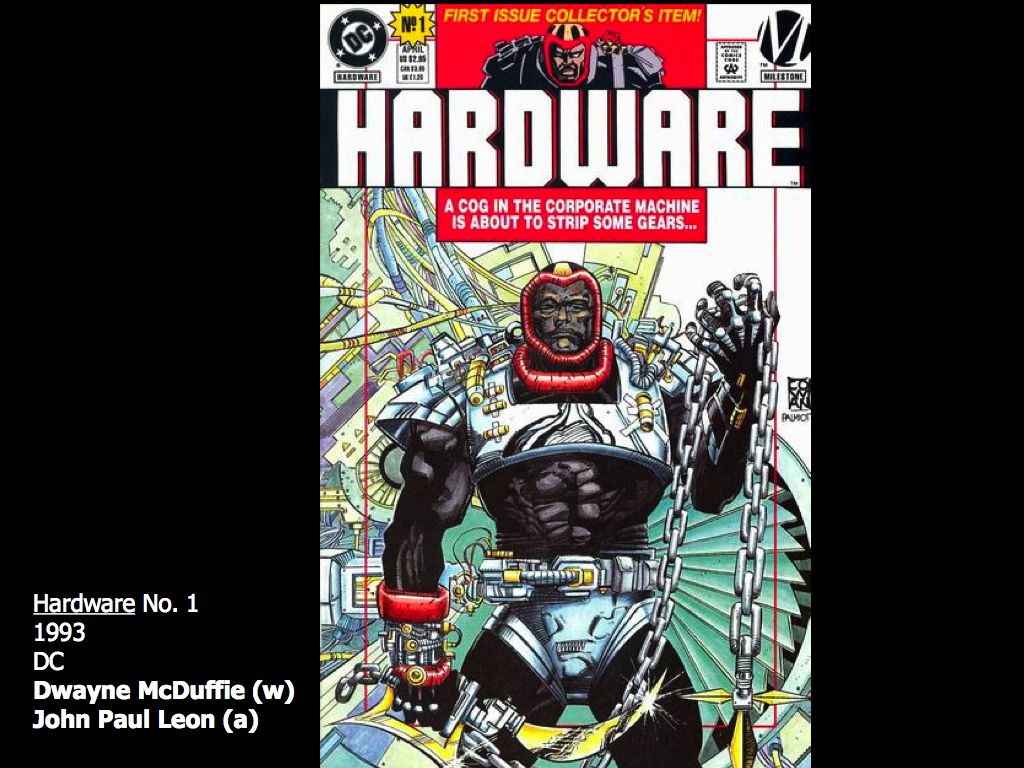This image presents a first edition collector's item of the DC comic book, Hardware. The cover features issue number one, prominently showcasing the title "Hardware" in a stylized white font on a black band background, positioned in the center of the top third of the cover. Below the title, the tagline "A cog in the corporate machine is about to strip some gears" appears in white text on a red background.

Dominating the cover is the illustration of an extremely muscular man integrated with machine components. He wears a tight-fitting black bodysuit adorned with metallic armor, including a silvery crop top and metal shorts. In one hand, he wields a technologically advanced scimitar, while the other hand grips a long chain link mace with sharp, angled blades.

The background features a primarily mechanical aesthetic, possibly depicting a jet engine, reinforcing the concept of him being part of and confronting the machine. The cover is centered within the image, and in the lower left-hand corner, identifying information details the comic's specifics: Hardware, issue number one from 1993, published by DC. The creators are listed as Dwayne McDuffie (W for writer) and John Paul Leon (A for artist).

This detailed depiction not only highlights the collectible nature of this comic book but also serves as an effective advertisement or product listing for enthusiasts and collectors.